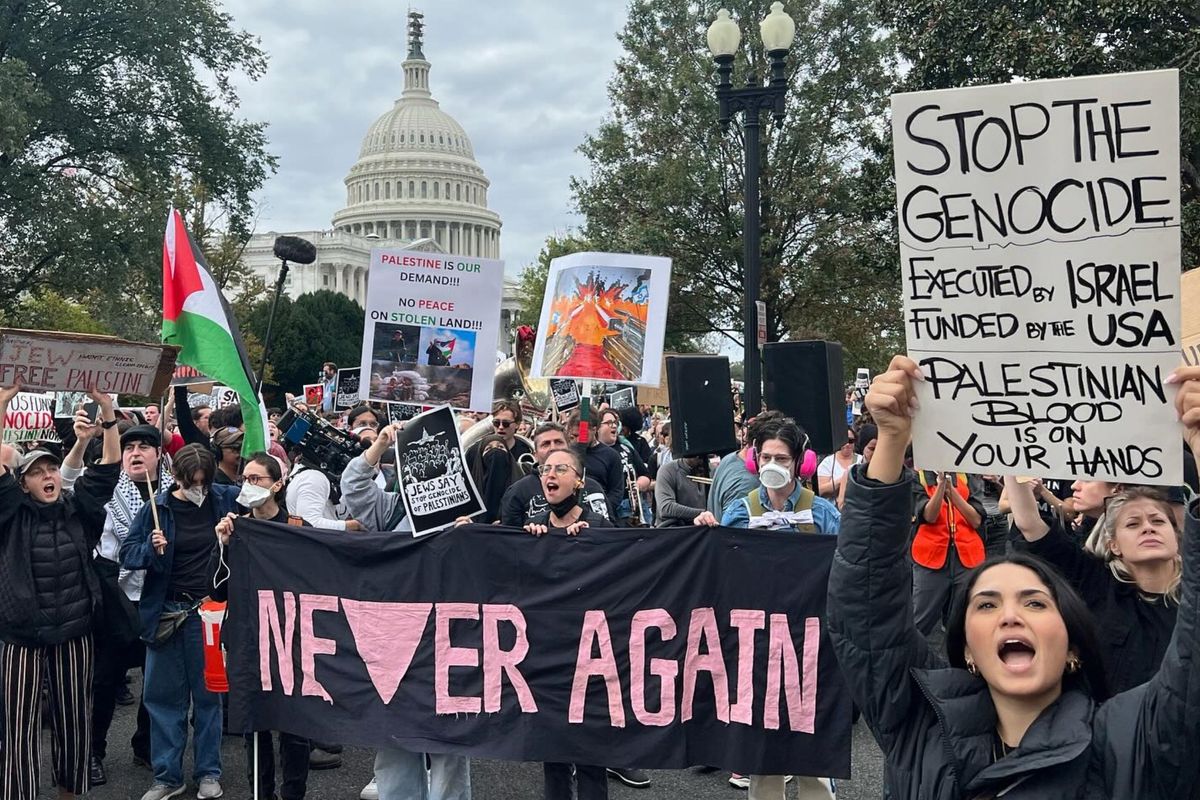In the foreground of this detailed photograph, a large group of demonstrators is gathered for a protest in front of the Capitol building in Washington, D.C., which is visible in the background, partially obscured by trees on the left and right sides. A prominent black street lamp with double lanterns stands on the left side of the image. Among the crowd, a woman on the far right holds a white sign with black text stating, "Stop the genocide executed by Israel funded by the USA. Palestinian blood is on your hands." 

Centrally, several people are holding a black banner with a pink upside-down triangle symbol and the words "Never Again" in bold pink letters. Just left of the center, another sign reads, "Palestine is our demand. No peace on stolen land." Further left, a Palestinian flag is being waved, and a white sign with black writing appears, stating "Jew Free Palestine." Some demonstrators are wearing masks and shouting, adding to the charged atmosphere. The scene is punctuated with various other signs, all contributing to the palpable intensity of the protest.